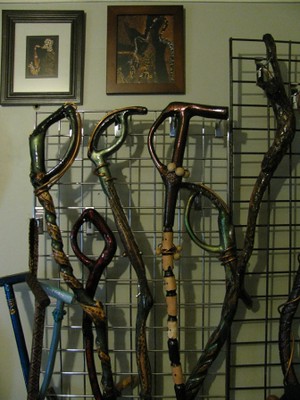The photograph captures an intriguing interior scene showcasing a collection of canes displayed on a metallic mesh grid against a grayish-green wall. In the top left corner, two framed images adorn the wall. The left frame, with a black outer rim, features a small image of a character holding a base kind of instrument to their lips, oriented to the left side. The right frame, with a brown rim, contains a dark and ambiguous portrait composed of light browns, dark browns, and blacks.

The prominent feature of the image is the array of canes, approximately nine in total, varying in design, color, and material. These canes are intricately designed and appear polished, indicating their decorative nature. They range from polished wooden canes to metal ones with unique handles. Notably, there is a cane with a copper-like handle and a bamboo base with dark brown segments, a shiny dark green cane with a swirled gold and black end, and blue metal canes positioned on the far left. These canes, which could be of cultural significance or specialized design, add a distinct character to the photograph, showcasing craftsmanship and diversity in their construction.